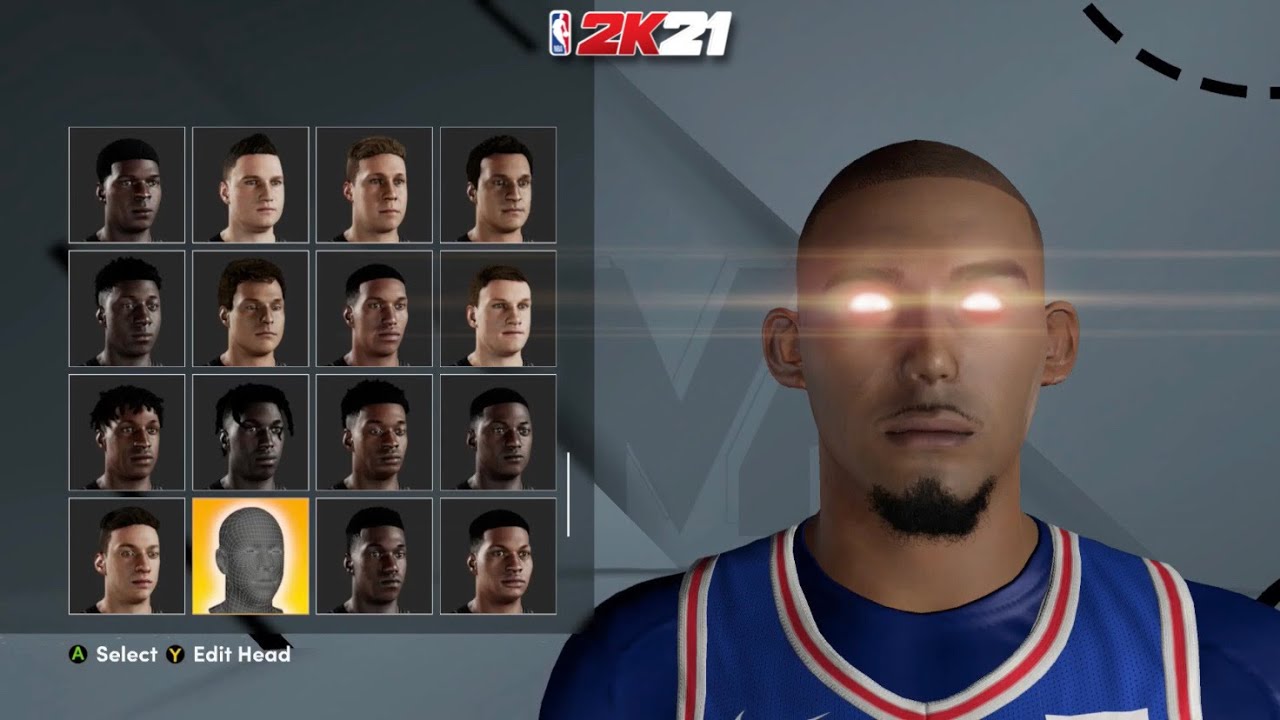The image features a predominantly grey background with subtle dashed lines in the upper right-hand corner. At the center, there's a prominent basketball logo displaying "2K" in bold red letters alongside "21" in white. To the left, there is a darker grey square or rectangle, containing 16 different faces, one of which is highlighted in yellow. Below the highlighted face, a small black circle with a green "A" denotes the word "Select," while another small black circle with a yellow "Y" indicates "Edit Head."

On the right-hand side of the image, there's a player depicted with unique, glowing white eyes that lack visible pupils. He is dressed in a blue and red jersey with a matching blue undershirt. The player has a bit of a goatee and mustache and is portrayed as a Black man with slightly protruding ears. The overall image is visually stimulating, combining various design elements to create a cohesive representation likely associated with a basketball video game interface.